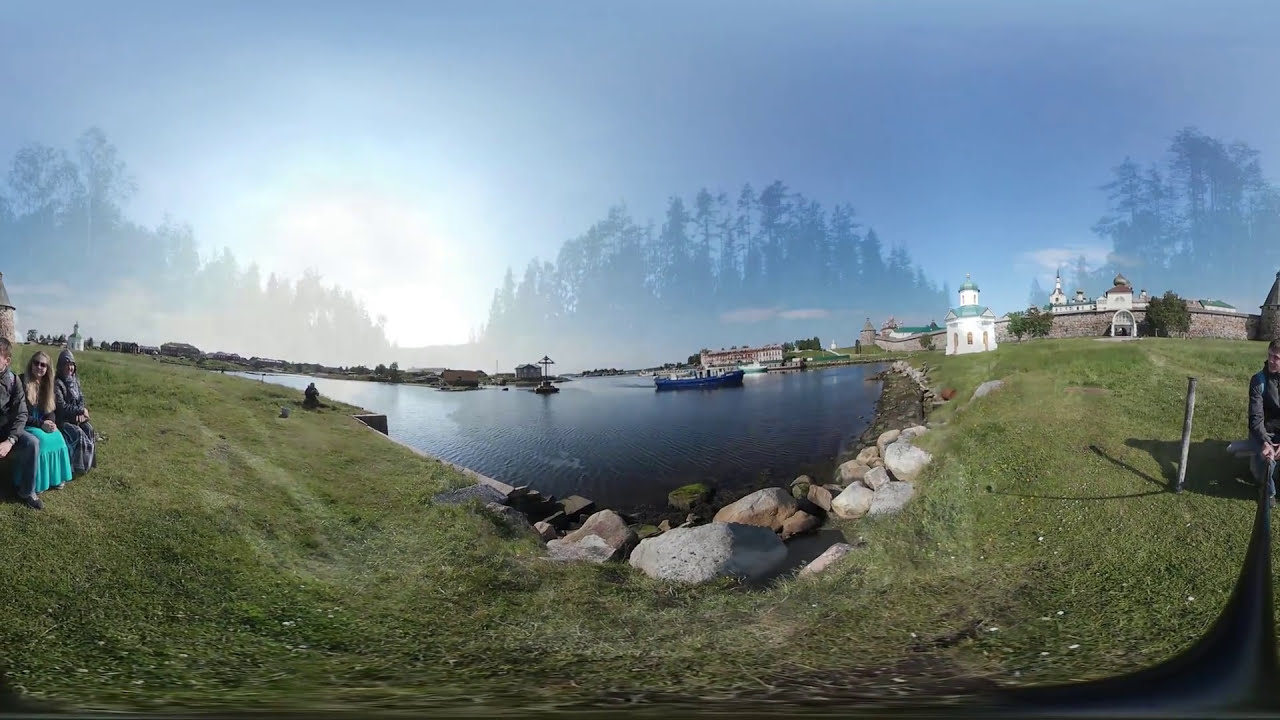This photograph, captured with a wide-angle lens and a selfie stick, features a man sitting on a bench who is looking away from the camera. The scene encompasses a picturesque, historic area that evokes an ancient, medieval, or Renaissance-era village. The foreground shows a vibrant green grassy area, bordered by gray and light brown stones that separate it from a body of water—be it a lake, pond, or river. In the water, there is a long boat that draws attention in the middle of the frame.

To the left side of the photograph, three people are seated on a bench, enjoying the view. Some are sitting directly on the grass or on stones. The background displays an idyllic, misty forest setting, potentially enhanced with photoshop, revealing a small temple or chapel amidst the trees. Alongside the water, one can see various older buildings, suggesting this is a historic site. Large rocks and boulders line the water's edge, and the sunlight casts a warm glow over the entire area, enhancing the serene and nostalgic atmosphere.